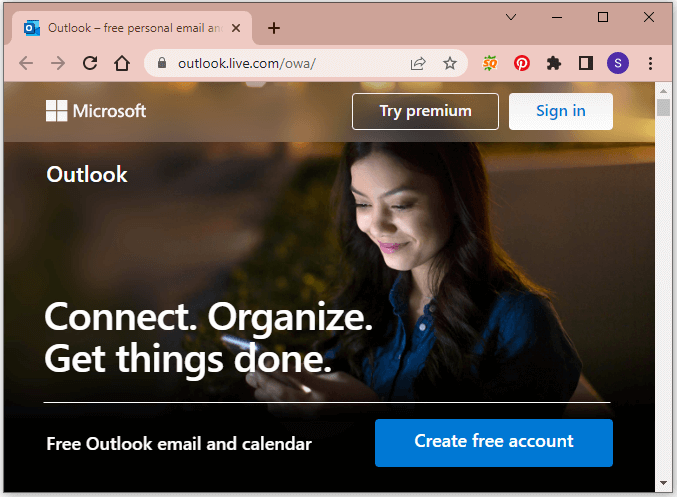This screenshot features a webpage design dominated by brown and pink tones, showcasing the Outlook interface. At the top, the browser tab displays with a blue icon, followed by the text "Outlook - Free Personal Email" in black. The search bar reads "Outlook.live.com/owha/." Below this, the Microsoft logo appears with the company name in white. To its right, a white button with blue text reads "Try Premium," adjacent to another button with a white background and blue letters that says "Sign In."

The main section of the page features an image of a woman with dark hair, dressed in a blue shirt. She appears to be in her late 30s or early 40s and is engrossed in looking down at a device, likely a phone, held in her hands. This photo is positioned with her face towards the left side of the frame.

Overlaid on the image, on the left side in white text, is the word "Outlook." Centrally positioned over her shirt in large white letters are the words "Connect. Organize. Get things done." Below this tagline, the text "Free Outlook Email and Calendar" is displayed. On the right-hand side, a prominent blue button invites users with the text "Create Free Account."